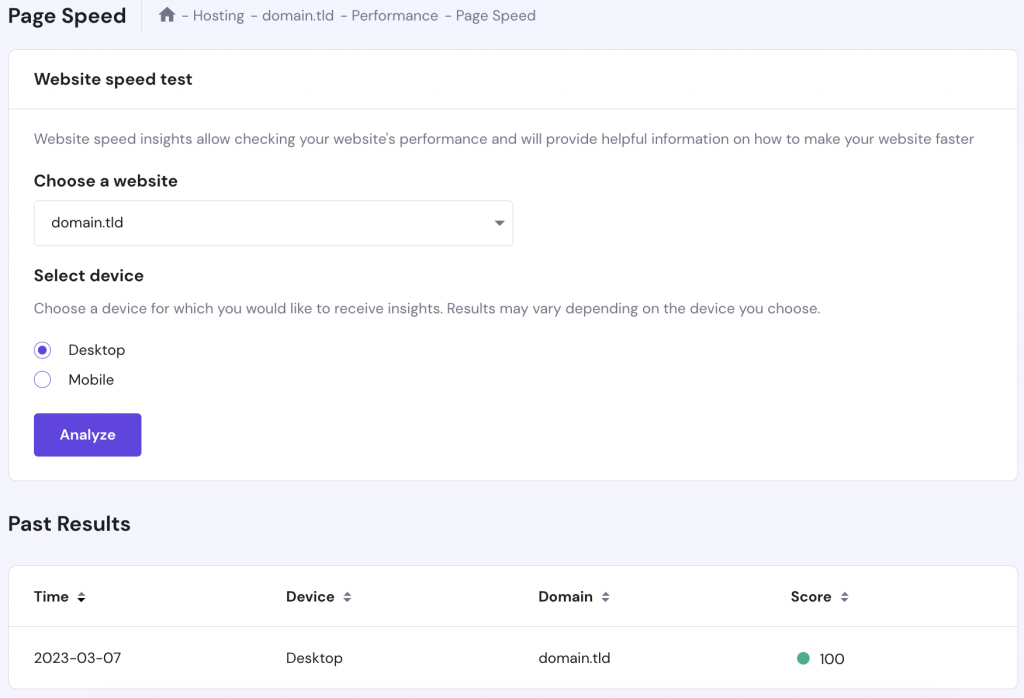The image captures a screenshot of a page speed test tool, presented in a portrait orientation with a gray border surrounding two prominent white boxes. The overall layout resembles a computer screen display, being wider than it is tall. At the top left corner, black text reads "Page Speed," followed by a subtle divider and a series of navigation links, including icons and labels for "Home," "Hosting," "Domain TLD," "Performance," and "Page Speed."

Below, a central white rectangular box with rounded corners contains detailed information and interactive elements. It starts with the headline "Website Test Speed" accompanied by a thin divider. The subsequent text explains: "Website speed insights allow checking your website's performance and provide helpful information on how to make your website faster."

A notable black section within the box invites users to "Choose Your Website," followed by a dropdown menu displaying "domain.TLD." Beneath this, an option labeled "Select Device" prompts users to choose a device type for which they want performance insights. Radio buttons for "Desktop" and "Mobile" are provided, with "Desktop" pre-selected and highlighted in purple, while "Mobile" remains unselected.

Towards the bottom of the box, a prominent purple button with white text reads "Analyze." Below this, a separate section is dedicated to displaying past test results.